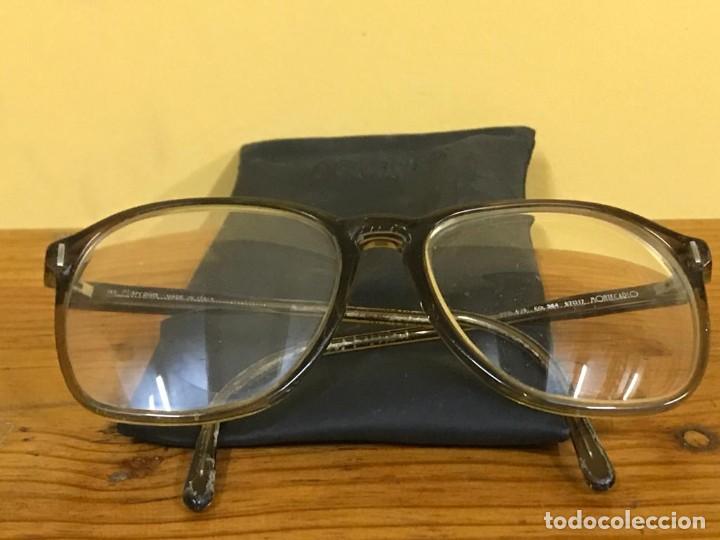A pair of eyeglasses with black and dark brown frames is showcased resting on a glossy black satiny pouch atop a wooden tabletop with noticeable horizontal wood grain. The lenses are clear, with a somewhat rectangular yet round shape, reflecting a light source from above. The wall in the background is a warm, inviting yellow or beige, enhancing the contrast with the black pouch. The eyeglass frames feature white writing on the inside, while the bottom right corner of the image displays the text "Todo Collection" in white, adding a branded touch to the scene. The overall setting suggests the photo was taken indoors, possibly in a cozy home environment.